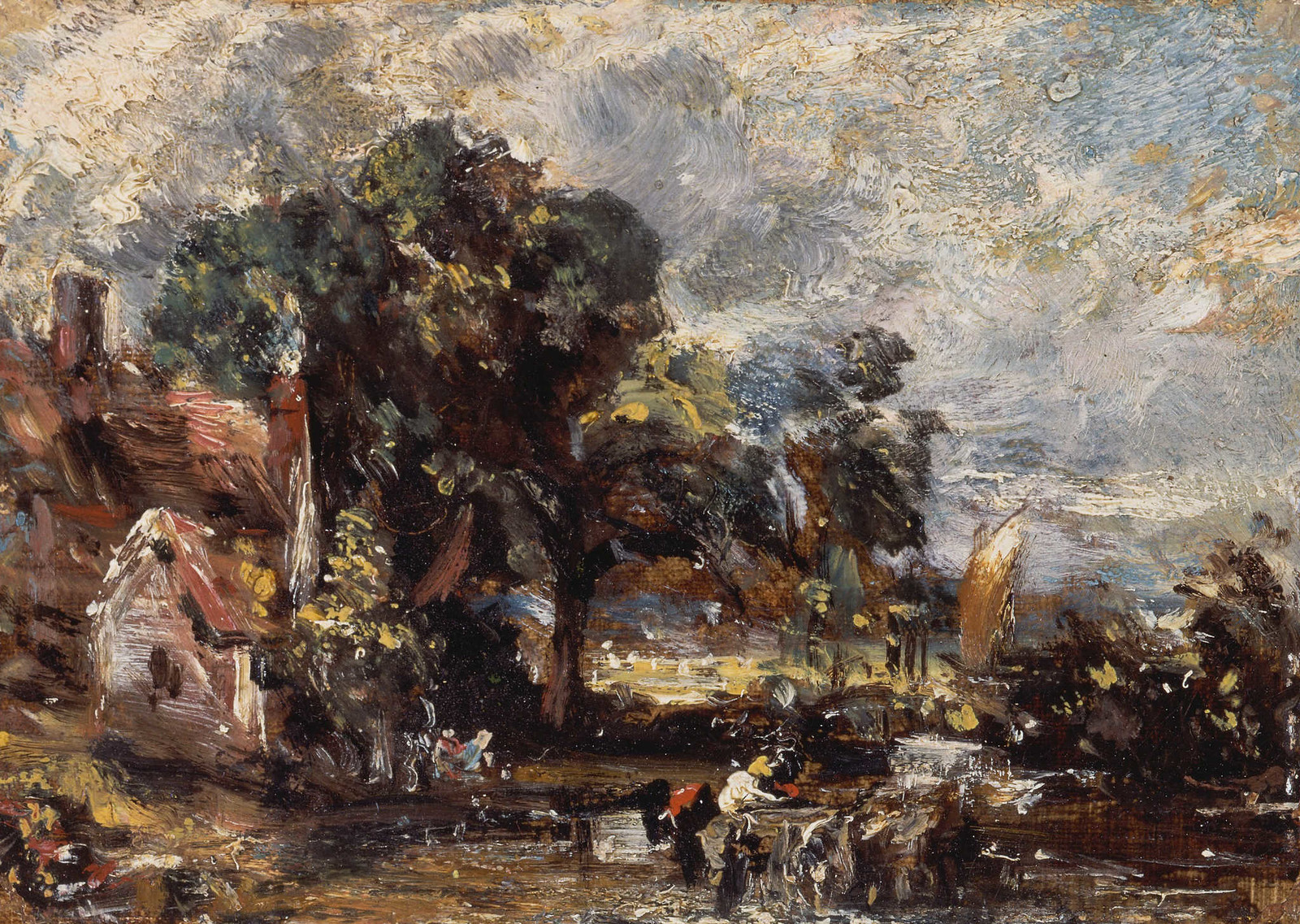An evocative oil painting with a dark, foreboding atmosphere, characterized by a turbulent sky filled with swirling grey clouds. Dominating the center of the composition is a large, gnarled oak tree, its branches sprawling across the canvas. Nestled in the lower left corner is a small, indistinguishable cottage, blending into the shadows. To the right, indistinct figures add a sense of movement and mystery, contributing to the overall busyness of the scene. 

On the left side of the painting, the faint outline of what appears to be a chimney suggests a larger building in the background. Closer inspection reveals what seems to be people or figures on the front lawn, with a pine tree nearby, possibly adorned with colorful decorations. Beneath the sprawling branches of the oak tree, a distant meadow or park comes into view. Here, ethereal white figures, perhaps dressed in elegant white gowns, populate a meticulously mowed lawn. This painting is rich in detail yet challenging to interpret, inviting viewers to delve into its complexities and find their own meaning.